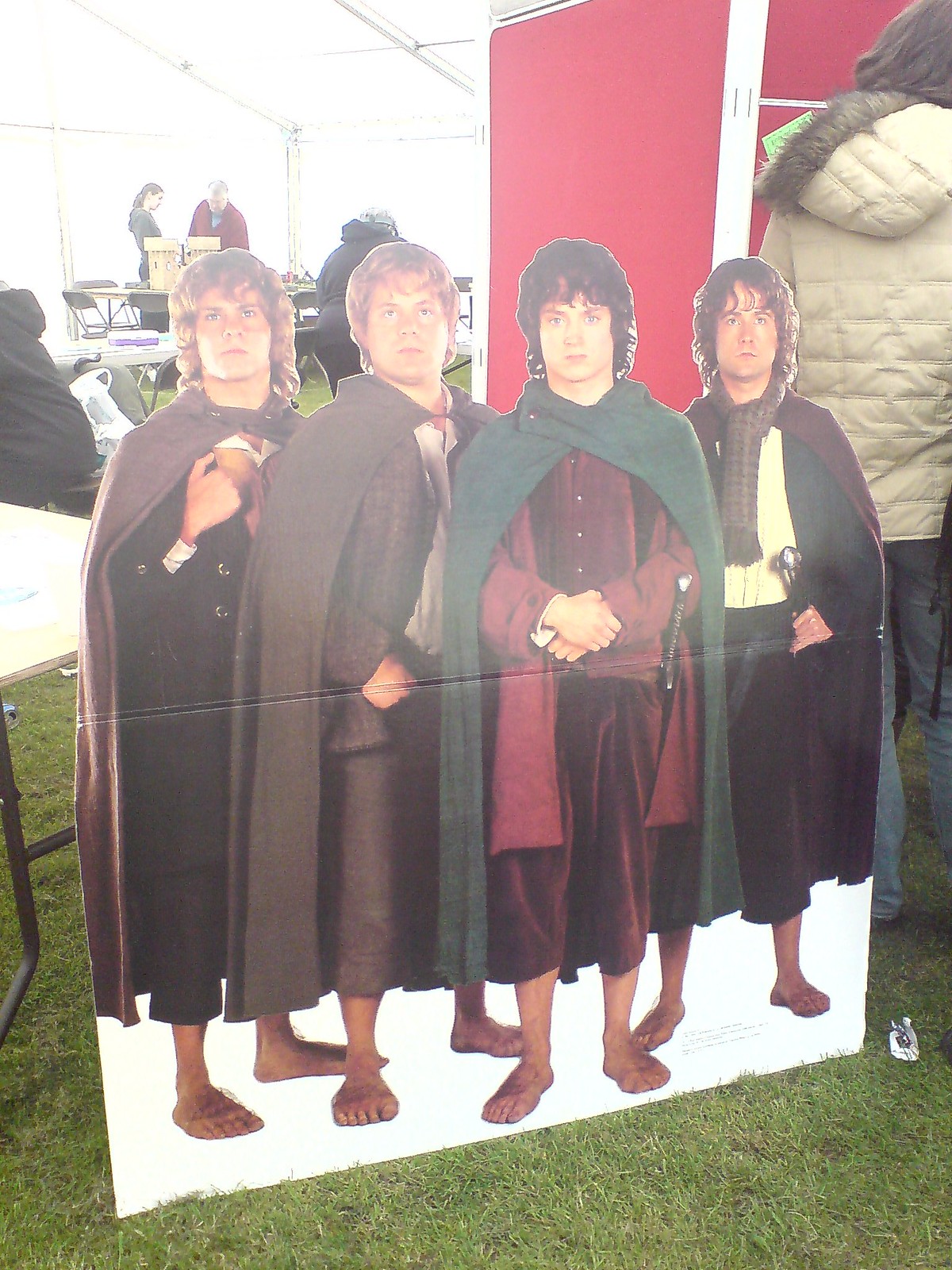The image depicts a detailed cardboard cutout poster of the four hobbit characters from the Lord of the Rings movie series, standing prominently on a patch of green grass. The cutouts, representing Samwise Gamgee and his fellow hobbits, are adorned in their signature medieval cloaks and attire, complete with their large, distinctive bare feet. Each hobbit varies slightly in appearance: from left to right, one wears a brown cloak with a black outfit, the next in another brown cloak with a brown outfit, followed by a character in a green cloak with a red jacket and knee-length pants, and finally, another in a brown cloak potentially wielding a sword hilt. The cutouts are strategically placed to give the illusion that the hobbits are present at the scene.

In the background, under what appears to be a large event tent, a woman in a light beige, fur-collared winter jacket and blue jeans stands facing away from the camera, near a red and white cabinet or trailer. The setting is bustling, with more people visible in the distance around tables and chairs, possibly preparing for or attending an event.

The area is well-lit, suggesting strong lighting often seen in tented events. Overall, the image conveys a lively scene where the beloved characters from Lord of the Rings are brought to life amidst a dynamic, real-world gathering.